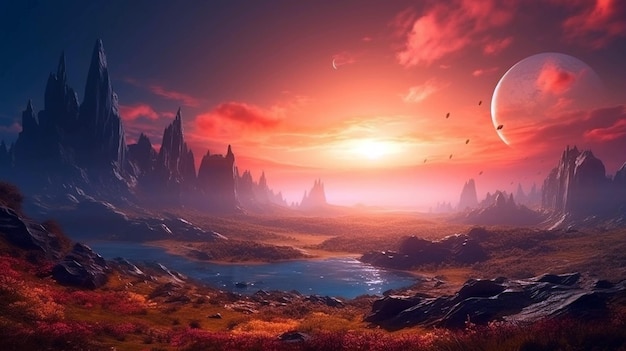This is an AI-generated image depicting an alien landscape, characterized by surreal and jagged rock formations that tower like spiny spires of varied heights. These dramatic peaks, arrayed sporadically across the scene, lack any flat surfaces and contribute to the overall sense of otherworldliness. In the foreground, a turquoise blue pond reflects the unique panorama, bordered by yellowish-green grass interspersed with small pink flowers and miniature versions of the tall formations. 

A bright, perhaps alien sun casts an ethereal light from the center of the sky, illuminating an orb on the far right that resembles a planet or moon. This scene is painted against a backdrop of a vivid blue sky streaked with wispy clouds enhanced by the warm, almost surreal colors of a setting or rising sun. The sun itself appears low on the horizon, casting a red-orange glow that adds to the picture's unearthly quality. Additionally, the sky features strange elliptical blobs, further enhancing the alien atmosphere. The combination of these elements forms a stunning visual that is unmistakably not of Earth.